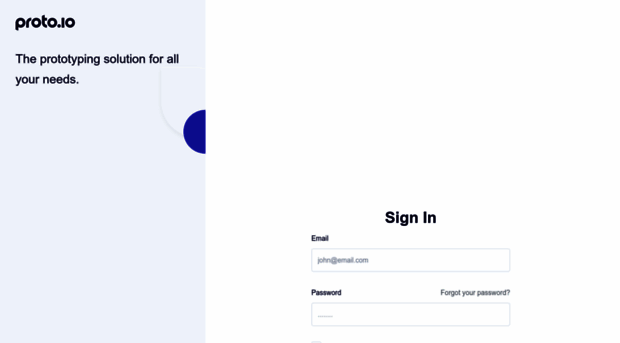The image showcases a sign-in page that has a clean, minimalist design with a primarily white background. The central focus is a large, light gray rectangle positioned on the left side of the page. Within this rectangle, there is a partially visible circle, suggesting an incomplete graphic element located slightly above the middle of the rectangle.

At the top-left corner of the image, the bolded black text "Proto.io" is prominently displayed, followed by a tagline in smaller text: "The prototyping solution for all your needs." 

On the right side of the page, near the bottom right, the sign-in area is clearly defined. The word "Sign-In" is bolded in black font, directly above two fields for user input. The first field, labeled "Email" in small text on the left, contains a placeholder example that reads "john@email.com." Below this, a similar setup exists for the "Password" field, both labeled in black font. To the right of the password field, a "Forgot your password?" link is available. 

Overall, the image captures a segment of a user-friendly sign-in interface, emphasizing clear text and a straightforward layout for ease of use.